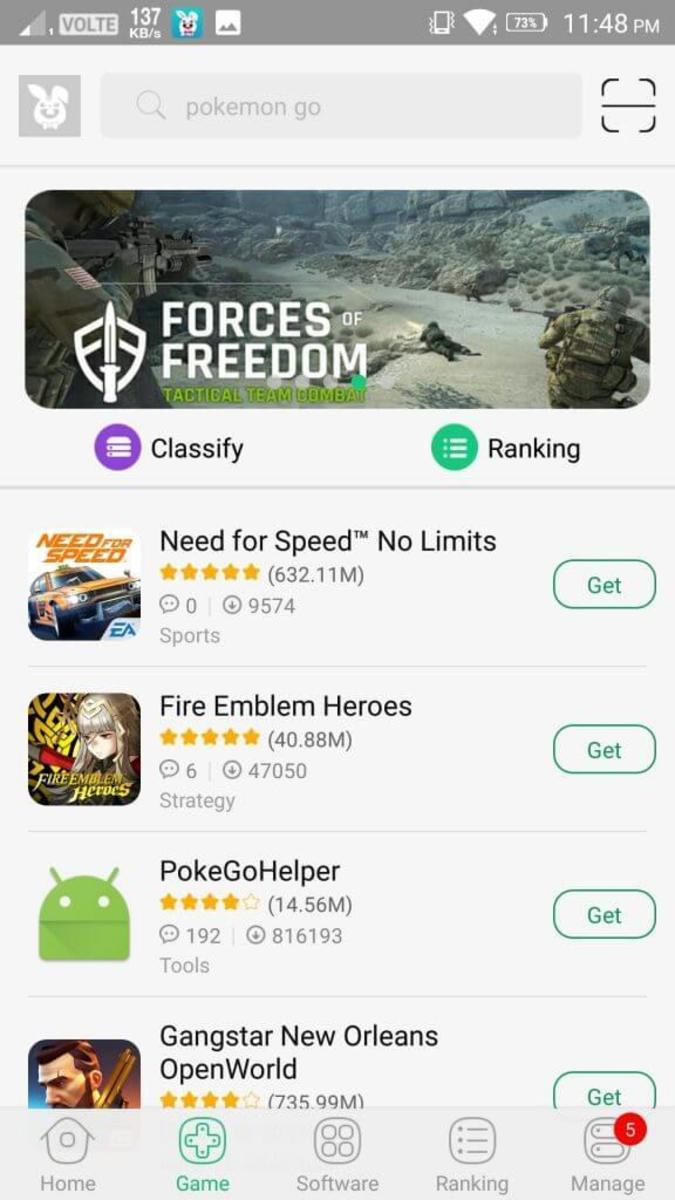The mobile screenshot showcases an app store interface, though it is not the Apple App Store. The top part of the image features a visually appealing background, above which a centered search bar appears. The search bar contains the text "Pokémon Go." To the left of this search box is a gray square decorated with an image of bunny ears, while on the far right is an icon resembling a scan image.

Beneath the search bar, a prominent header displays an image related to the game "Forces of Freedom," portraying dynamic gameplay. In the bottom left corner of this header image, a shield and knife logo is visible, accompanied by the game's title, "Forces of Freedom," in bold, large white letters. Toward the bottom center of the screenshot, a series of dots appear, with the fourth dot highlighted, indicating the image is the fourth in a photo carousel.

Below the "Forces of Freedom" image, two separate labels are positioned. On the bottom left, a purple icon labeled "Classify" is visible, and on the bottom right, a green circular icon labeled "Ranking" is present. Following this section is a vertical list showcasing various apps and games.

The first game in the list is "Need for Speed No Limits," featuring a thumbnail on the left, with its title, ratings, and category information positioned to the right. Adjacent to this information, on the far right, there is a "Get" button. Additional apps and games follow in the same vertical format, creating a comprehensive view of available options.